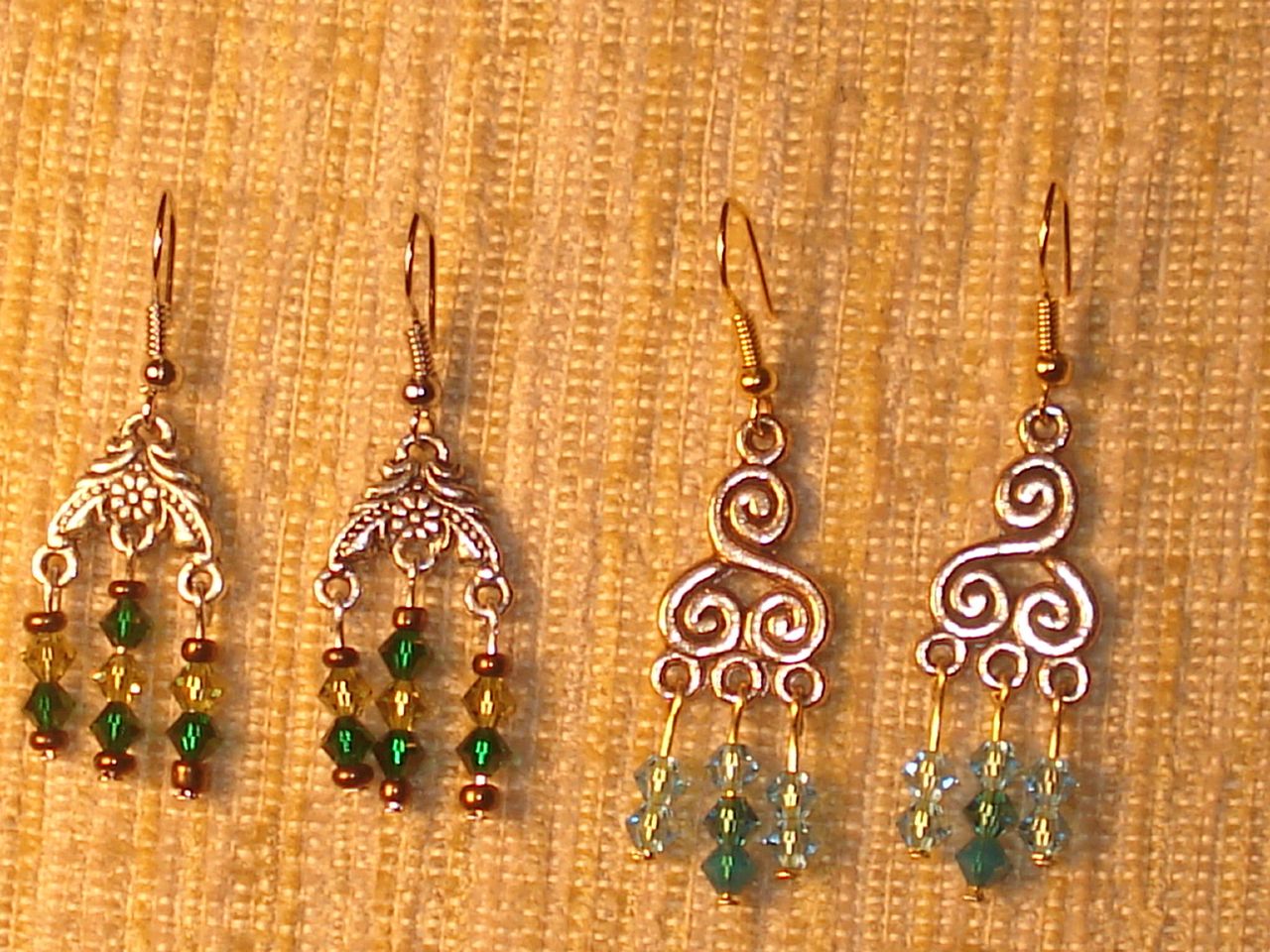This image features two pairs of vintage-inspired, gold dangle earrings displayed on a beige or gold-colored textured fabric, possibly cotton or burlap. Both pairs of earrings have gold hooks and intricate metal designs from which three sets of beads hang. 

The pair on the left has a floral motif with delicate filigree that prominently showcases a small flower in the center, accompanied by six decorative dots on either side. Each of its three dangling strands features a sequence of beads: a round bronze bead, a diamond-shaped yellow bead, a green bead, and another round bronze bead, all connected by wire pins.

The pair on the right exhibits a Celtic-inspired scroll design, resembling swirling clouds. The beads on these earrings are primarily aqua and turquoise, arranged as two beads on the first strand, three lighter and darker aqua beads on the middle strand, and two aqua beads on the third strand. This detailed arrangement offers a harmonious blend of colors and shapes, enhancing the earrings' vintage charm.